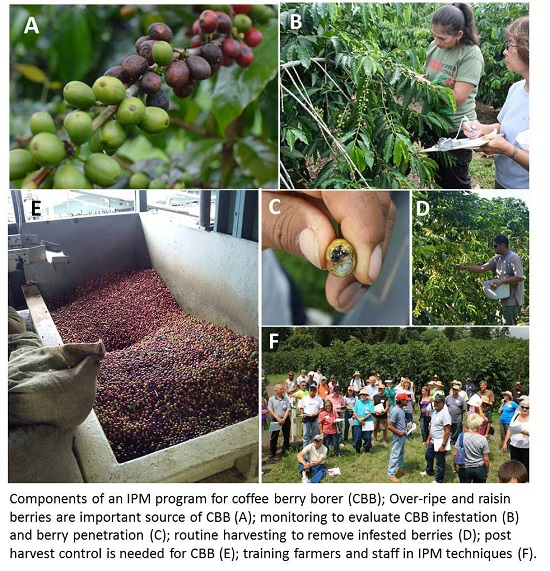The image is an educational guide about coffee, consisting of six distinct pictures labeled A through F. Picture A displays ripe and unripe coffee beans, which are initially green. Picture B shows two individuals, a woman in white and another in green, picking coffee beans from green plants. Picture C reveals a close-up of a coffee bean's interior, held in someone's hand. Picture D captures a man in a gray shirt and sunglasses, picking coffee beans with a white bucket. Picture E features a white bin filled with harvested coffee beans of varying shades of brown, gray, and tan. Picture F depicts a large group of people gathered on a grassy lawn, likely part of an educational session about coffee; the attendees are dressed in various colors, some wearing hats. Below these images, detailed text explains the Integrated Pest Management (IPM) program for Coffee Berry Borer (CBB). It highlights the importance of over-ripe and raisin berries as CBB sources, monitoring CBB infestations and berry penetration, routine harvesting to remove infested berries, post-harvest control, and training farmers and staff in IPM techniques.